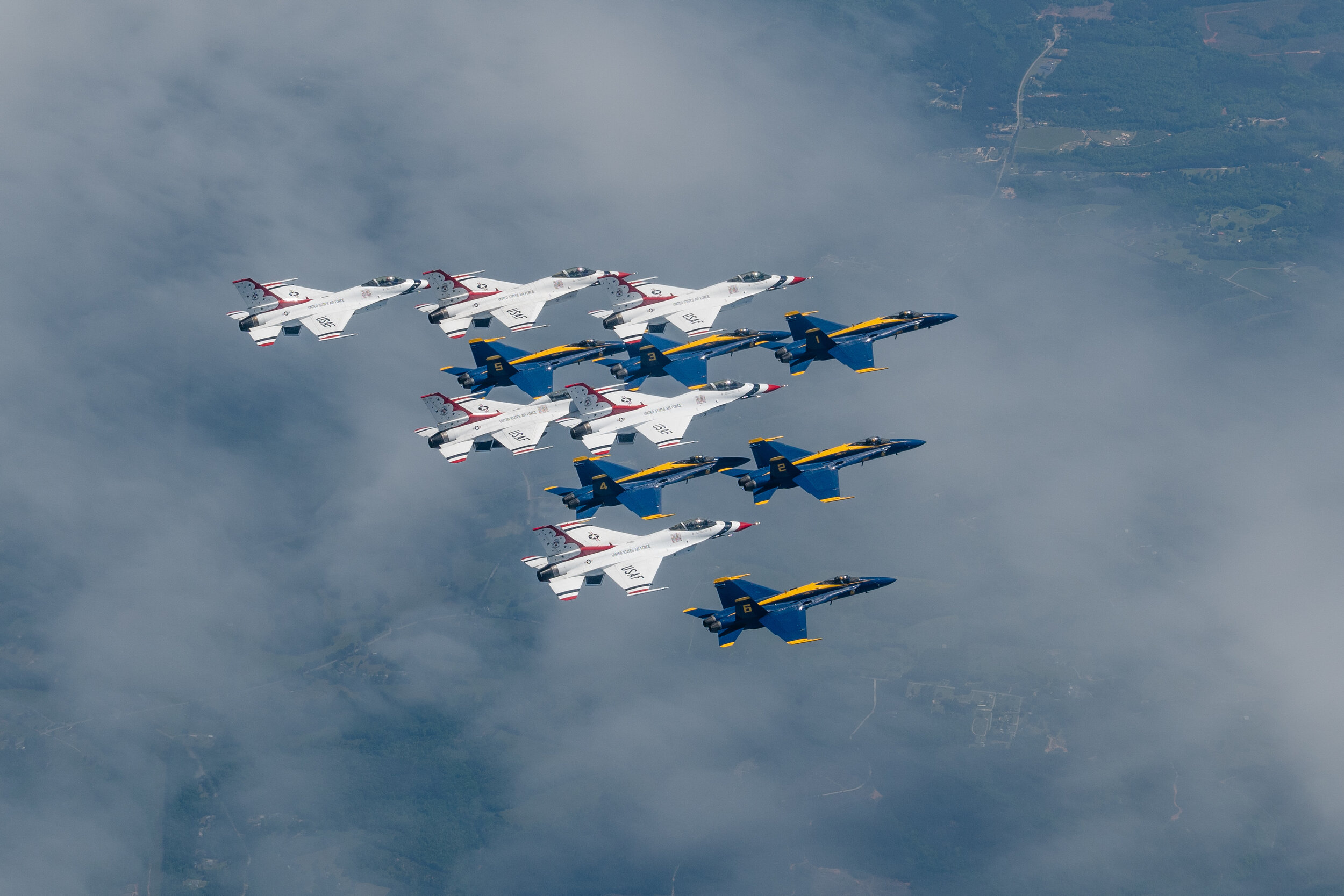The photograph captures a squadron of fighter jets in an intricate triangular formation, appearing almost as if viewed from above. This aerial shot showcases the jets flying closely together, their wings nearly parallel, against a backdrop of a hazy sky with light clouds below them. The jets come in two distinct types: blue-bodied with golden-yellow highlights and white with red accents. The formation consists of a total of twelve jets, evenly split between the two types. The leading jet is a blue one, and the pattern alternates with blue and white jets interspersed throughout the triangle. Below the jets, faint glimpses of green fields and small trees are visible through the clouds, adding depth to the composition.